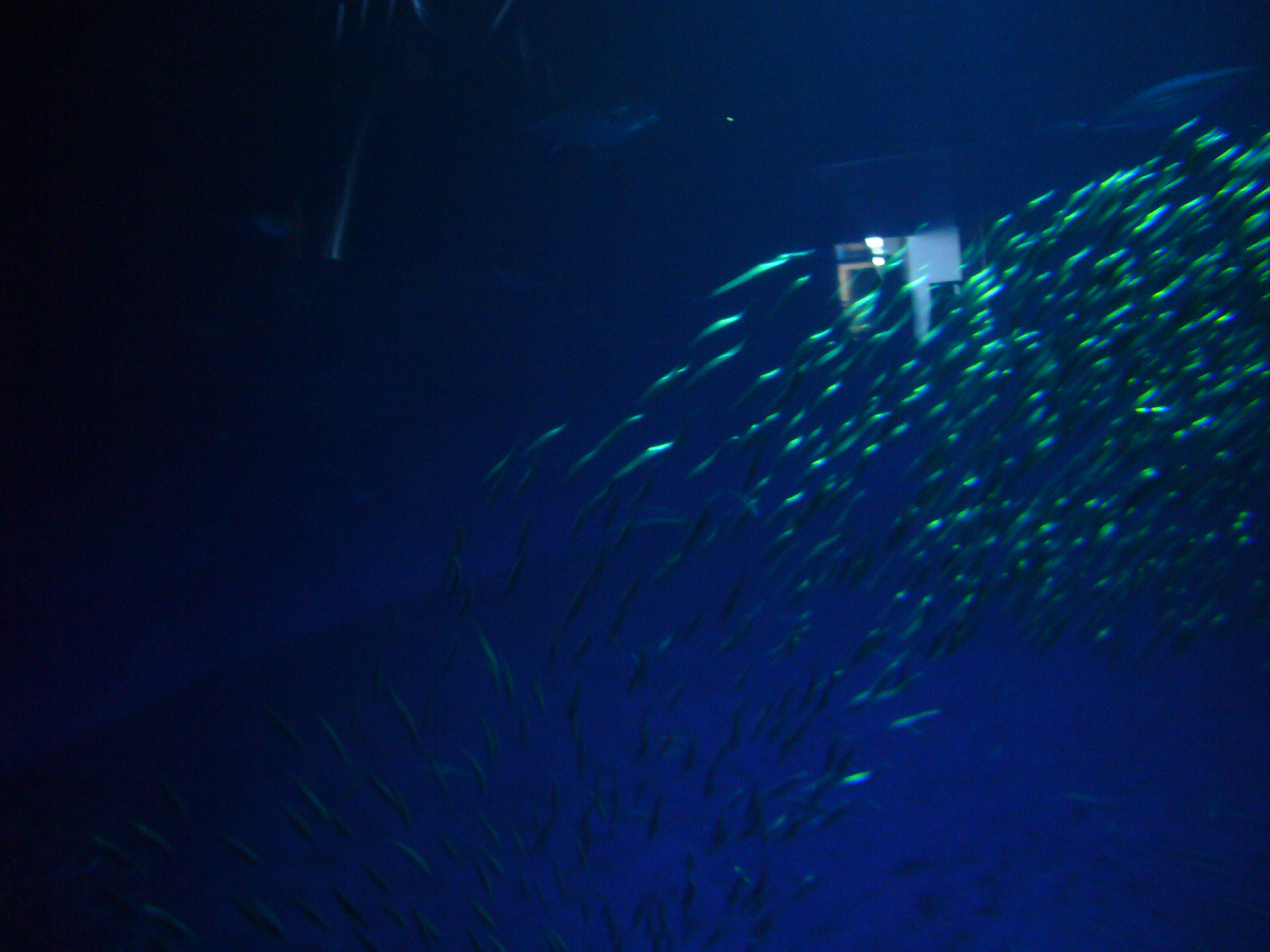This underwater photograph showcases the mesmerizing scene of a large school of small fish in motion. The image captures the stark contrast between darkness and light, indicative of deeper waters, with the left side nearly enveloped in blackness and the right side illuminated by faintly filtering light. The overall blue hue of the water enhances the aquatic atmosphere, occasionally interrupted by yellowish or greenish tints from the fish. The fish, possibly numbering in the thousands, appear to be caught in the midst of dynamic movement, swimming from the bottom left to the top right of the frame. The blurriness created by their rapid motion makes them somewhat indistinct, adding a mystique to their identity. This suggests an aquarium or a vast, contained water tank environment. The chaotic splash-like marks around the fish further accentuate the sense of motion and the underwater setting. This vivid snapshot effectively conveys the frenetic energy and fluid beauty of an underwater ecosystem.